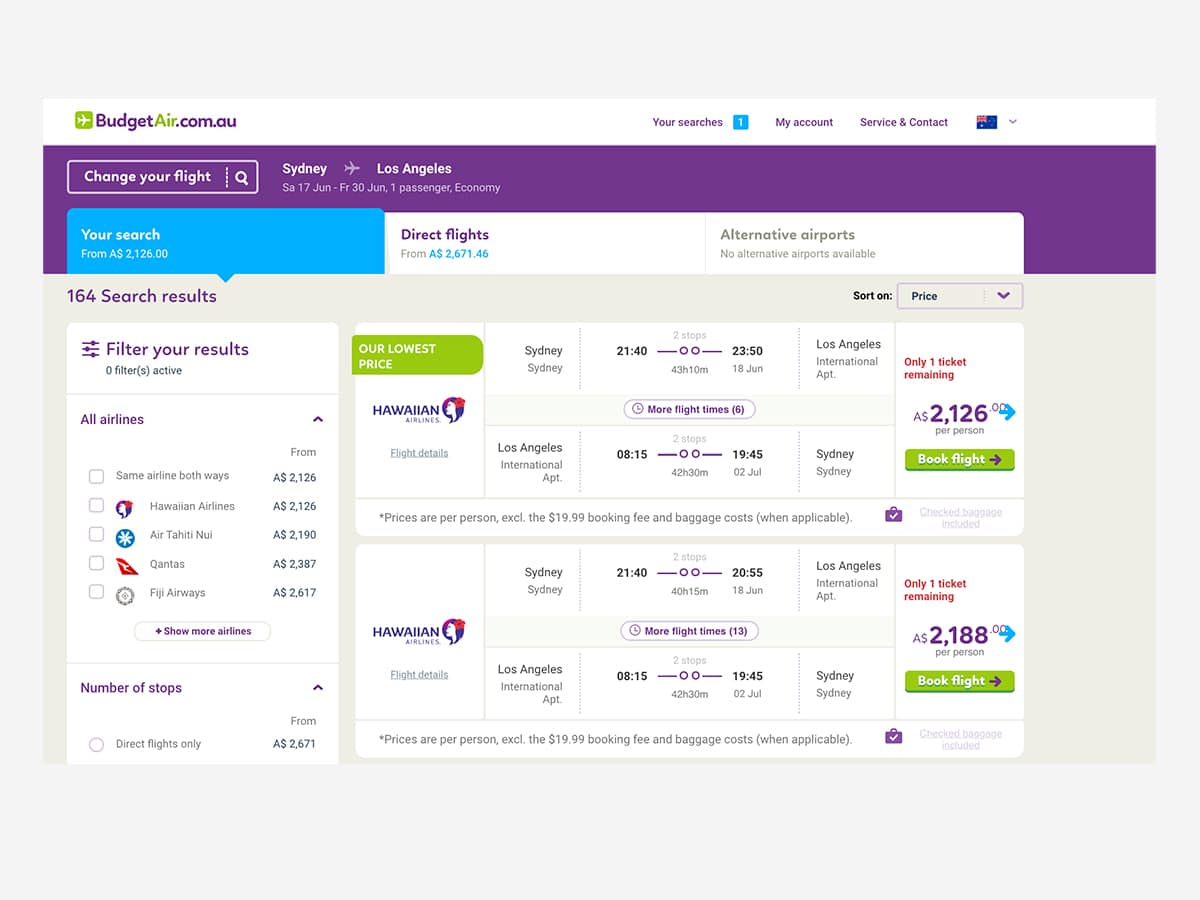The image is a vibrant and colorful web page from BudgetAir's Australian site, budgetair.com.au. The background features an array of colors including purples, greens, blues, whites, and grays. The "Budget" in the domain name is written in purple, "Air" in green, and ".com.au" in purple. The web page includes a graphic of an airplane within a square design.

At the top of the page, there is a purple banner displaying "Your searches" in purple text, next to a blue square box with the number one, indicating perhaps a step or prioritized search result. The "My account" and "Service and contact" links are also written in purple. Additionally, there is an Australian flag displayed prominently.

The top banner of the page is purple, displaying the message "Change your flight to Sydney to Los Angeles." Below this banner, it details a search with the query resulting in a price of 2,126 AUD for direct flights, with options for alternative airports.

A green bar across the page highlights "Our lowest price, Hawaiian Airlines." The flight details indicated involve departures from Sydney to Los Angeles with a fare of 2,126 AUD per person. There is another flight option listed at 2,188 AUD per person. Both of these options are in red text, emphasizing that only one ticket remains available for each flight.

On the left side of the page, there is a list of airlines, though the specific names are not detailed in the description. The layout and colorful design emphasize ease of use and navigability for users looking to book flights.